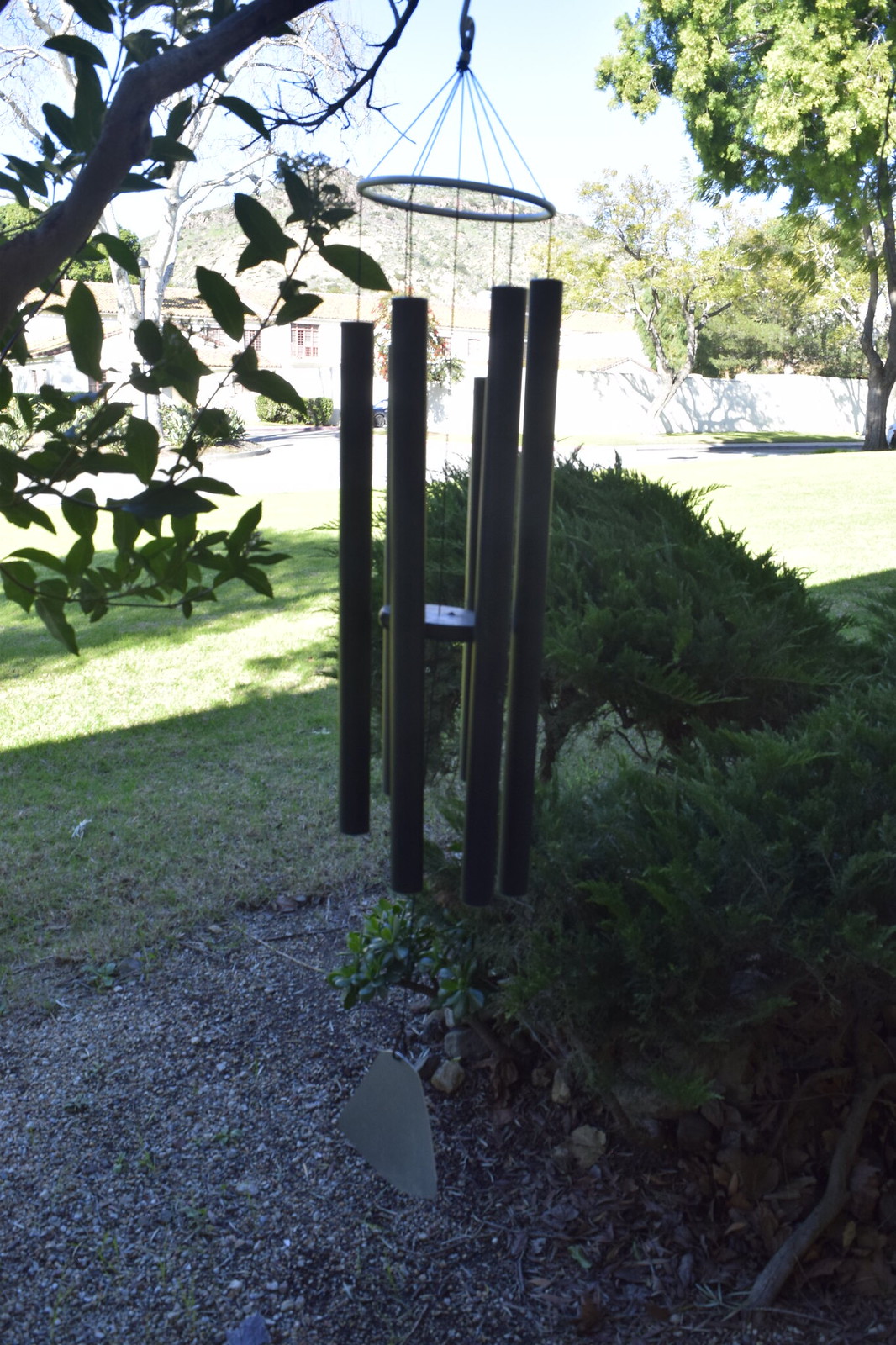This outdoor image features a set of wind chimes hanging elegantly from a circular ring at the top, suspended by strings. The wind chimes consist of five to six clear tubular cylinders, which are made of metal, and they surround a thicker, black circular disc in the center that they strike against to produce sound. The scene is set amidst a lush garden where the vibrant green grass captures the sunlight, creating a bright contrast with the darker shade spots beneath the foliage. A variety of plant life is visible: a tree with light and dark green leaves stands to the far right, while on the left, a branch and a few leaves protrude into view. The ground below the chimes is neatly landscaped with gray decorative gravel, home to several types of bushes. In the background, a white wall or fence clearly delineates the boundary of a house, adding a hint of structure to this tranquil outdoor setting.